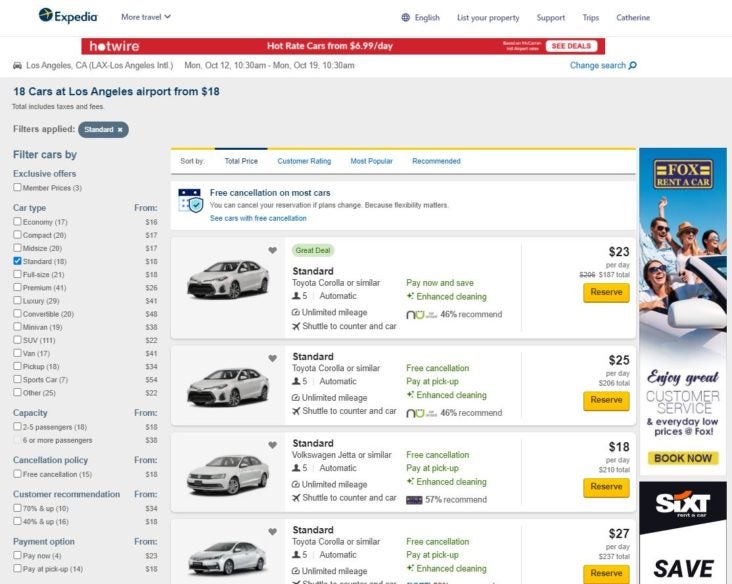Expedia Car Rental Options at Los Angeles Airport:

Displayed are 18 car rental options starting at $18. Featured prominently are four standard cars, primarily in white or silver hues. Three Toyota models are priced between $23 and $27, and a Volkswagen is available for the lowest rate at $18. The top-listed Toyota Corolla is highlighted as a "Great Deal" and includes green text indicating benefits such as "Pay Now" and "Free Cancellation." Key features like price details, reserve buttons, and car images enhance user experience. For those planning a trip, the interface is straightforward and includes a handy filter button for customized searches.